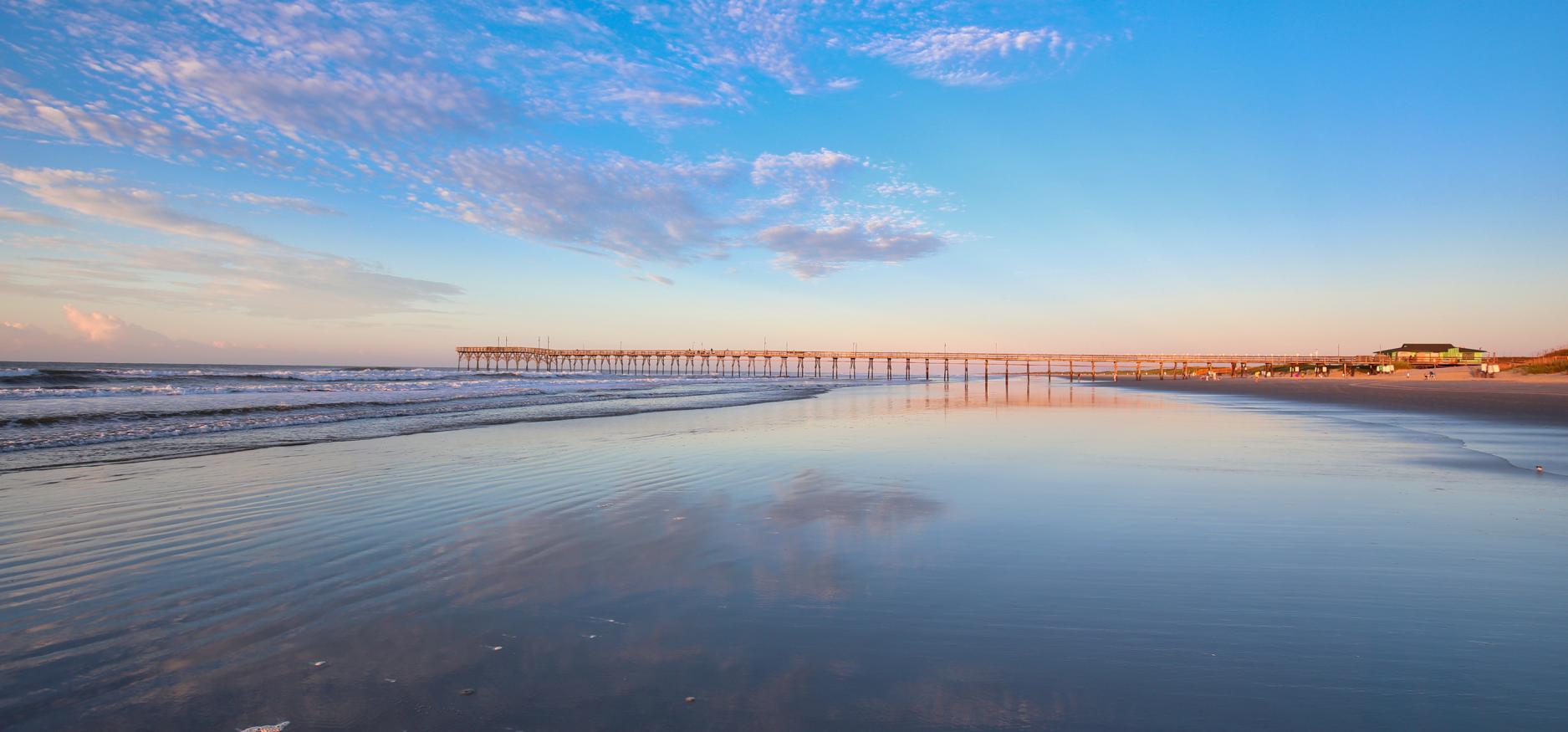This photograph captures an early morning scene at a beach, characterized by a clear blue sky with a few wispy clouds. In the foreground, the sandy shore glistens with the remnants of the receding tide, and gentle waves roll towards the ocean. Dominating the landscape is a long pier, extending from a building on the right-hand side of the image and reaching out into the shimmering water. There are faint silhouettes of people that appear to be walking along the pier in the distance. The serene and quiet atmosphere of the beach—evident from the lack of visible crowds—invites thoughts of a tranquil, picturesque locale perfect for fishing or a reflective stroll.